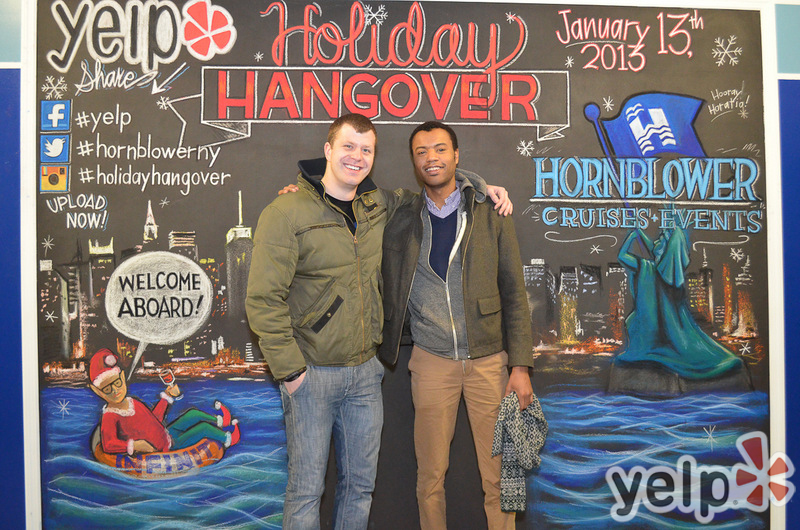The image captures two men posing in front of a detailed promotional board for an event. The man on the left is wearing a green puff jacket with blue jeans and has his hands in his pockets. The other man, standing to the right, is dressed in a green jacket with a gray sweatshirt underneath and beige pants, holding a scarf in his hand. The board behind them showcases a vivid cityscape with buildings in the background and a stylized Statue of Liberty holding a blue flag on the right. In the foreground of the board is a body of water, where a man in green pants, red shoes, a red shirt, and a red cap with a white puffball is depicted floating on a life preserver.

Prominently displayed above the two men in red text are the words "Holiday Hangover," with the date "January 13, 2013" to its right. The board also features a series of hashtags and social media prompts, including "Yelp," "HornblowerNY," and "Holiday Hangover," with a call to "Upload Now." Below the date and event title is the text "Hornblower Cruises & Events," indicating the likely sponsor of the event. Additionally, there is an image of an elf holding a glass of wine, reinforcing the festive theme. Across the bottom of the board are symbols for social media platforms like Facebook and Twitter, along with the word "Yelp."